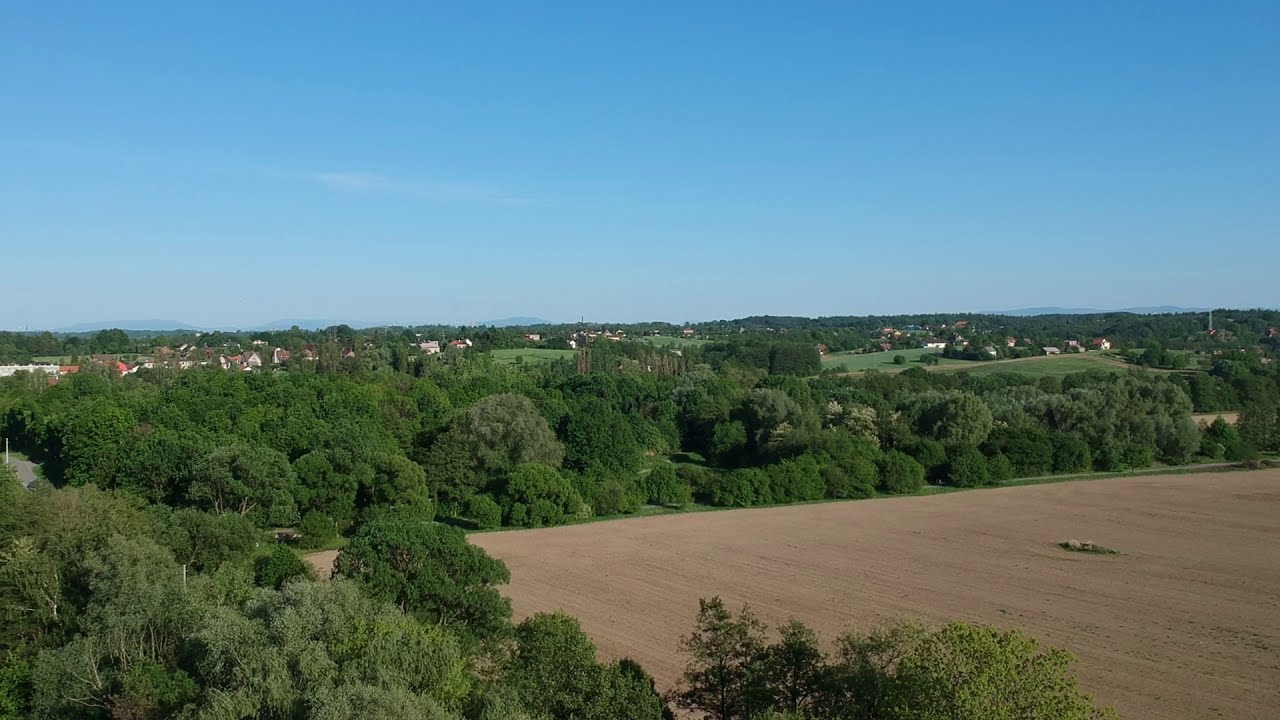The image captures a vast, lush landscape from an aerial perspective, showcasing a vibrant mix of natural and man-made elements. In the bottom right corner of the frame lies a freshly tilled rectangular farmland, featuring a light brown-tan color, indicative of recent agricultural activity. Surrounding this cultivated area are dense clusters of green, deciduous trees and verdant grass, creating a stark contrast against the plowed earth.

Extending from the periphery of the farmland towards the center of the image are more densely packed clusters of trees, giving way to a populated area that appears to be a town. The town is characterized by multiple buildings with distinct white walls and red roofs, primarily grouped in the middle center of the image. Further to the right, the buildings become more scattered, interspersed among additional green spaces, with a prominent tall white antenna marking the landscape.

In the background, rolling hills stretch across the horizon, adding to the picturesque quality of the scene. The sky above is a light blue, punctuated with sporadic, wispy white clouds, suggesting a clear, pleasant day, likely in spring. The overall flatness of the ground accentuates the vastness of the horizon, making for a harmonious blend of cultivated land, vibrant forest, and settled areas, all under a serene azure sky.